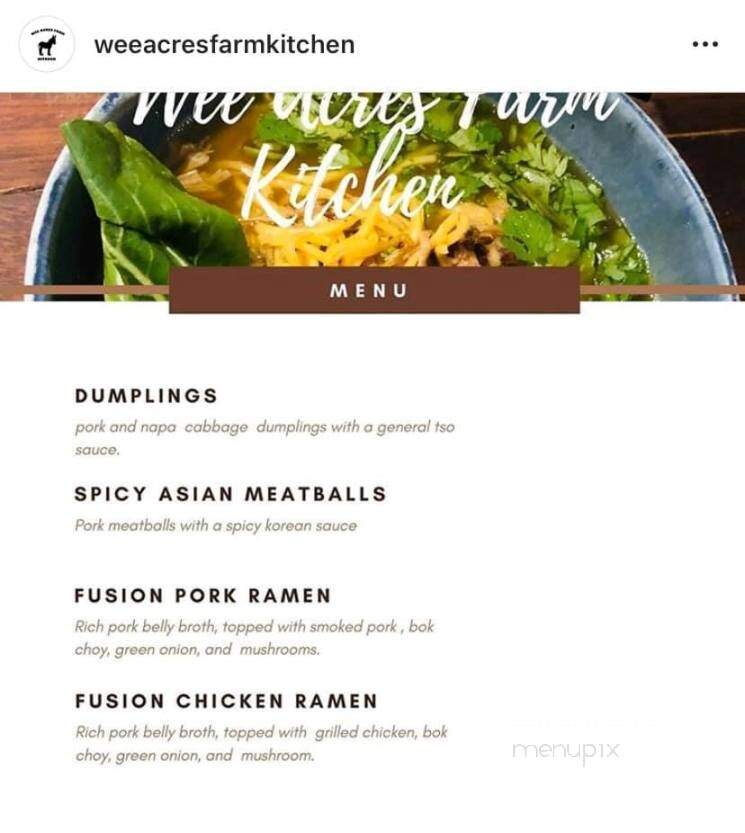The image features a detailed menu from "We Acres Farm Kitchen." In the top left corner, the silhouette of an animal resembling a horse or donkey, rendered in black, provides a rustic touch. Adjacent to the silhouette, in black text, is the establishment’s name: "We Acres Farm Kitchen."

Below this, a silver bowl is prominently displayed, containing a liquid base, with shredded cheese and green herbs generously sprinkled throughout. At the center of the bowl, a brown box with the word "Menu" in bold text draws attention.

The menu items are listed below in black capital letters, starting with:

1. **Dumplings**: Described as pork and Napa cabbage dumplings served with a flavorful General Tso sauce.
2. **Spicy Asian Meatballs**: These are pork meatballs accompanied by a spicy Korean sauce.
3. **Fusion Pork Ramen**: A rich pork belly broth forms the base, topped with smoked pork, bok choy, green onions, and mushrooms.
4. **Fusion Chicken Ramen**: This dish features a rich pork belly broth as well, but is topped with grilled chicken, bok choy, green onions, and mushrooms.

The image combines visual elements with descriptive text to provide a thorough overview of the available dishes at the "We Acres Farm Kitchen."